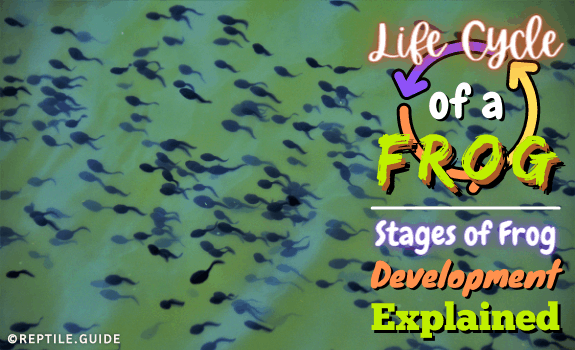The image is a rectangular graphic commonly used for websites or educational materials, depicting the life cycle of a frog. The background consists of greenish, brackish water interspersed with light blue hues, creating a natural setting through which numerous black tadpoles swim from right to left.

On the right-hand side of the image, occupying about one-third of the space from the top down, is a detailed heading. It begins with the phrase "Life Cycle" in white cursive with a red outline, followed by "of A" in white print underneath. Below this, in green print with an orange shadow, the word "Frog" stands out prominently. Behind this text, two arrows, one purple and one yellow, form a circular graphic representing continuous cycles.

A horizontal white line divides this section from the lower text, which reads "Stages of Frog" outlined in purple, "Development" in orange, and "Explained" in green. 

In the lower left corner, in white print, is a copyright symbol followed by "reptile.guide," indicating the source or owner of the image. The overall design combines various colors—white, orange, green, yellow, and purple—to highlight the key concepts and stages of frog development, making it a visually engaging educational tool.